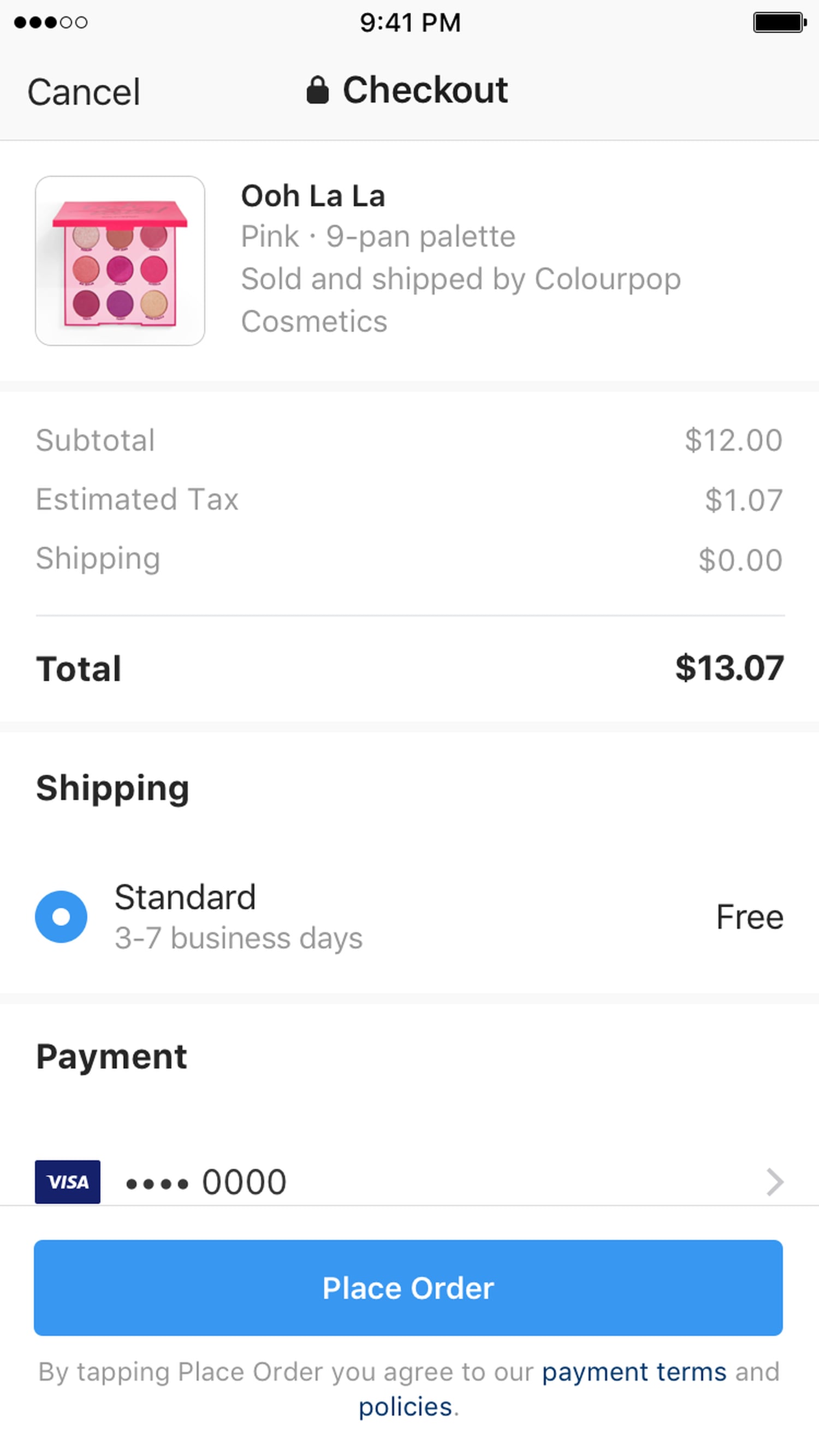The image displays a screenshot of a cell phone page, specifically the checkout section of an online purchase. At the top of the screen, there are five dots indicating the page markers, with three black dots on the left and two white dots on the right, suggesting that this is the third page in a sequence. The current time is displayed as 9:41 p.m., and the battery icon shows it is fully charged.

The screen header includes an option to cancel, with the main section titled "Ooh La La." Below the title is an image of a makeup palette, specifically a pink 9-pan eyeshadow palette, labeled as being sold and shipped by ColourPop Cosmetics.

Further down, the order summary details include:
- Subtotal: $12.00
- Estimated Tax: $1.07
- Shipping: Free

The total cost displayed is $13.07.

The shipping information notes that the standard delivery time is three to seven business days, with the cost being free, as indicated on the right-hand side.

In the payment section, there is an indication of the payment method, showing a Visa card number in a navy box with four black dots followed by "0000" for privacy. An arrow pointing to the right suggests additional options or details available.

At the bottom of the screen, there's a blue rectangular button with the text "Place Order." Beneath this button, a note states: "By tapping Place Order, you agree to your payment terms and policies."